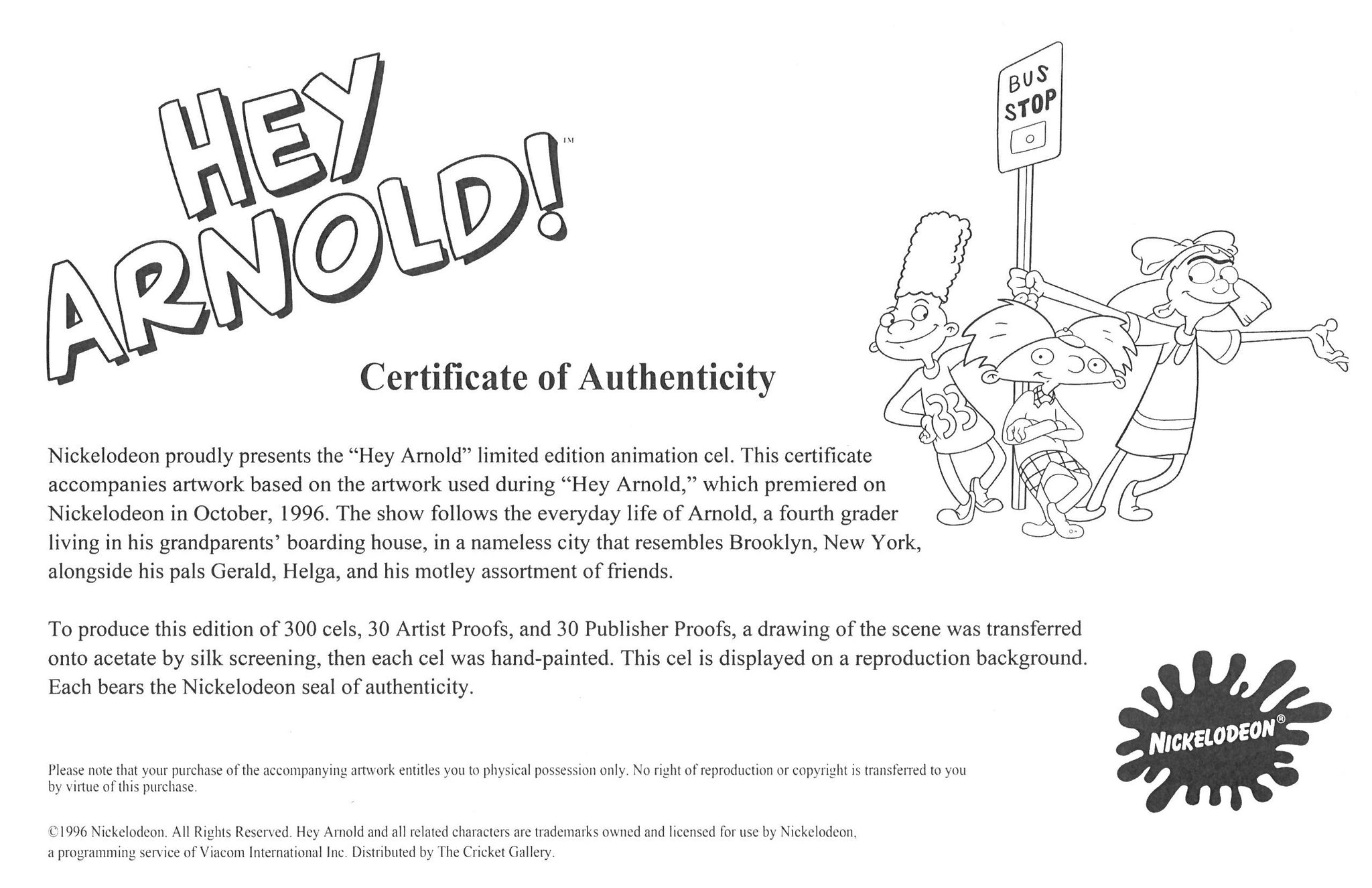This image depicts a Certificate of Authenticity for a Hey Arnold animation cell, presented in black and white. At the top center, the title "Certificate of Authenticity" is prominently displayed in bold, larger text. To the upper left, the iconic "Hey Arnold" logo appears in the show's signature font. On the right side of the image is an illustration featuring the characters Arnold, Gerald, and Helga from the Hey Arnold series, all in black and white. Arnold is seen leaning against a bus stop sign, with Gerald and Helga holding onto it as well. In the bottom right corner, the classic Nickelodeon splatter logo is present. Beneath the title, the text reads: "Nickelodeon proudly presents the Hey Arnold limited edition animation cell." It further explains that the certificate accompanies artwork modeled after scenes used in "Hey Arnold," which originally premiered on Nickelodeon in October 1996. Additional textual content provides details about the show's setting and character dynamics, along with the production process for the animation cells, noting that each cell was hand-painted and displayed on a reproduction background. The certificate concludes with a copyright notice and a disclaimer at the bottom.